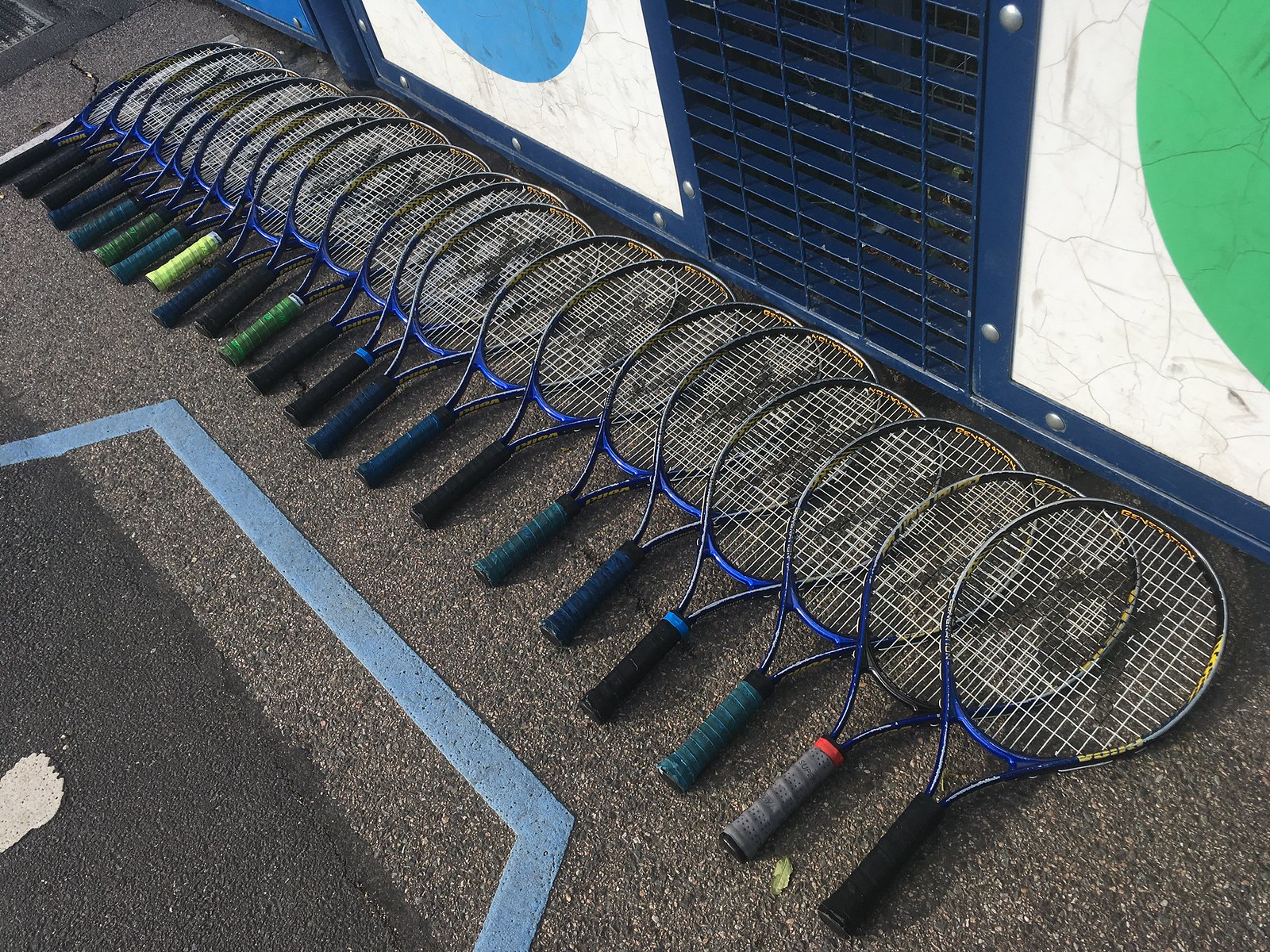The photograph displays a neat row of approximately two dozen blue tennis rackets, each with a triangular logo, arranged on a grey, asphalt-like surface that looks similar to the material used on tennis courts. The rackets overlap halfway with the next, creating a cascading effect, and a variety of colorful handles can be seen, predominantly dark but with unique red and yellow exceptions. This lineup is situated against a backdrop featuring a white wall exhibiting a patchy, marbled texture. On this wall are distinct blue and green circles, with blue on the left and green on the right. Additionally, the rackets are placed in front of a dark blue metal gate or grill, which allows some light to pass through its openings, suggesting the photograph was taken in daylight. A painted blue line forming a square is visible on the ground beneath the rackets.